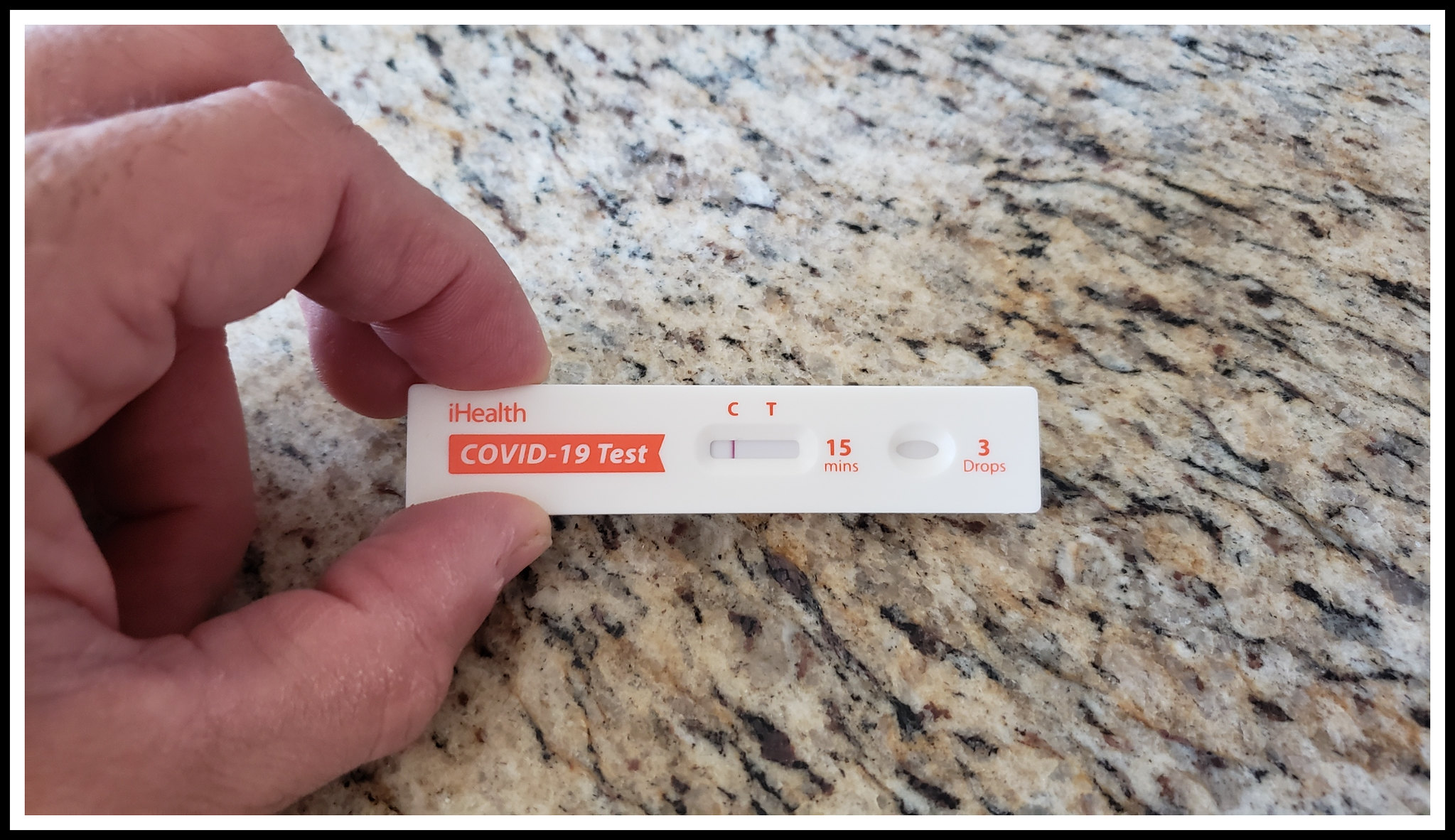The image showcases a COVID-19 test displayed prominently against a brown marble or granite countertop. The countertop exhibits a beautiful gradient pattern with tans, whites, and blacks blending seamlessly to create an intricate design. 

The COVID-19 test, branded as "iHealth," is centrally positioned within the frame. It is a white rectangular device featuring orange text reading "iHealth COVID-19 Test." The test has a small window through which two markers can be seen: a purple line under the "C" on the left side and instructions indicating "15 minutes" next to the window. Another smaller window beside this has the instruction "three drops" written next to it.

A man's hand is visible on the left side of the test, with the index finger and thumb grasping the device. His hand has noticeable hair on the knuckles and some dry skin around the thumb, adding a human element to the otherwise clinical test kit. The entire image is framed with a black border, with a thin white outline running inside the perimeter, emphasizing the rectangular format and directing focus to the central subject.